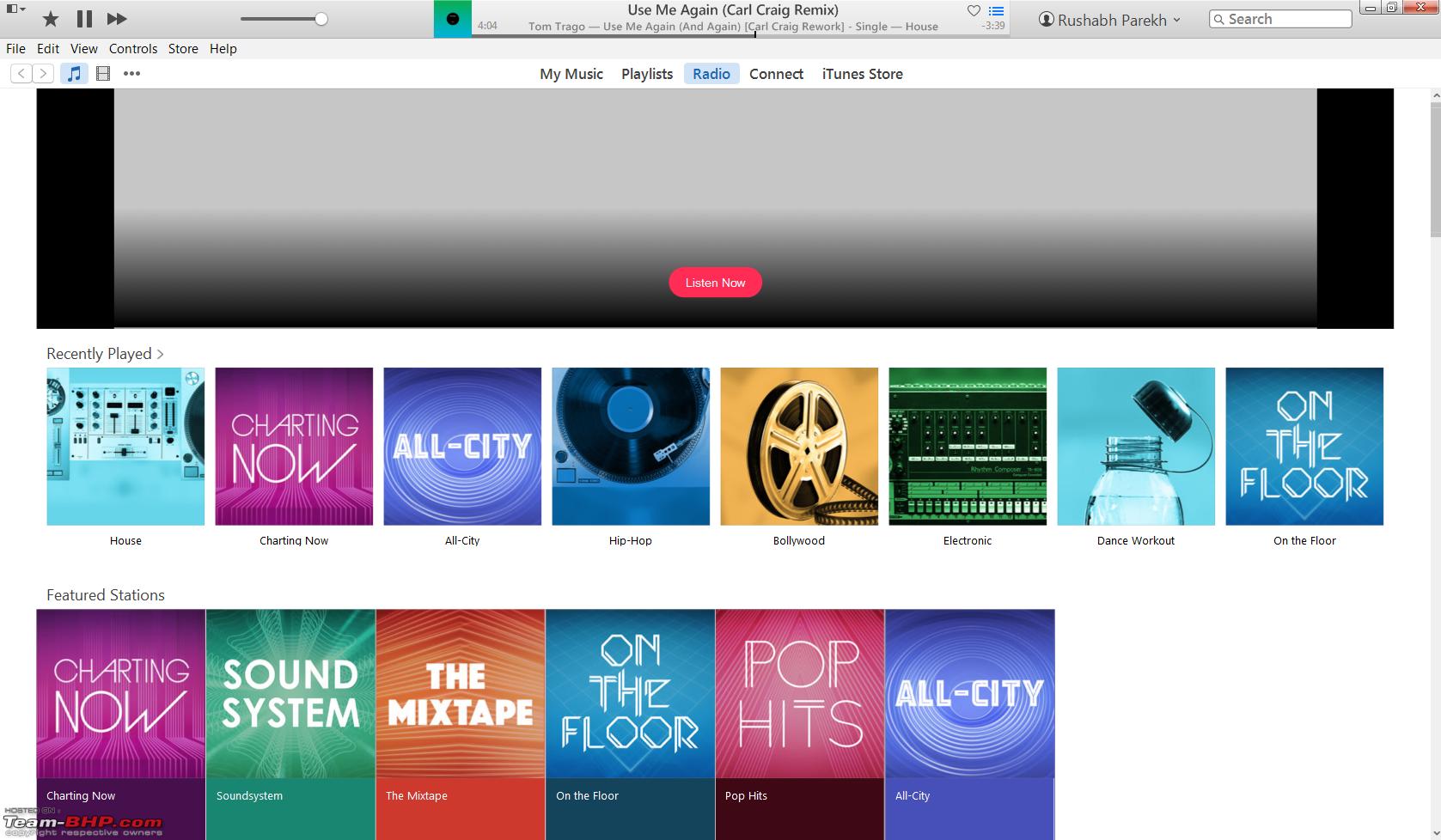**Detailed Caption:**

The image displays a music streaming website interface. At the top, there is a user interface section featuring a "Favorites" button, displayed as a star icon. The playback controls include a currently paused feature, a skip track button, and a volume control slider. The central part of the screen shows "Use Me Again (Carl Craig Remix)" as the currently playing track, with a progress timeline indicating four minutes remaining. The song is listed under the artist Tom Tragel as a single in the House genre.

The user, logged in as "rashfab perak," has options to change their account settings. A search bar is also available nearby. Navigation options include a minimize button, two boxes for window control, and a red "X" for closing the site.

Directly beneath the favorite star, there is a menu bar with options such as File, Edit, View, Control, Store, and Help. Below this, there are different sections including My Music, Playlist, Radio, Connect, and iTunes Store. The user is currently in the "Radio" section, highlighted in blue. This section features a "Recently Played" list displaying various album arts; one example is a stereo icon in blue labeled "House." There is also a "Charting Now" indicator in purple, displaying different genres like All City, Hip-Hop, Bollywood, Electric Dance, and Workout.

The "Listen Now" button is prominently displayed in red underneath the navigation sections. On the right side of the website, a scrollbar is visible for navigating the page vertically. The page layout and navigation controls suggest a user-friendly interface designed for easy access to music and personalized features.